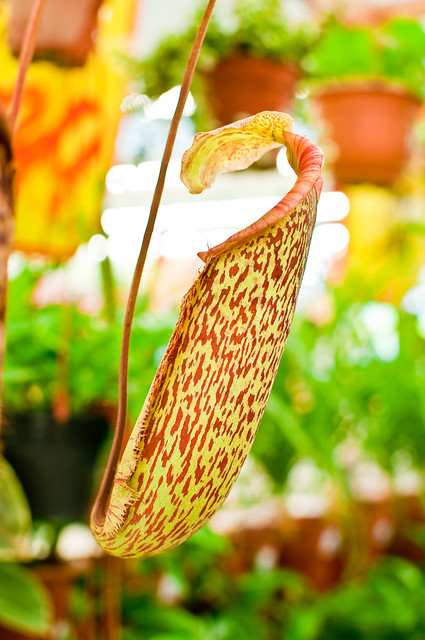In this vertically oriented image, the focal point is a striking leaf or blossom that dominates the forefront. The plant, possibly an unusual orchid, has a vividly colored, curved leaf with a stem descending into the frame. This leaf exhibits a prominent mix of yellow and orange hues with red blotches. Adjacent to this leaf is a smaller offshoot that's lighter in color. The background is blurred but discernible, featuring shelves filled with various green plants housed in terracotta and dark-colored pots, adding to the botanical setting's ambiance. The detailed textures and distinct coloration of the leaf or blossom make it the central subject against the backdrop of potted greenery.